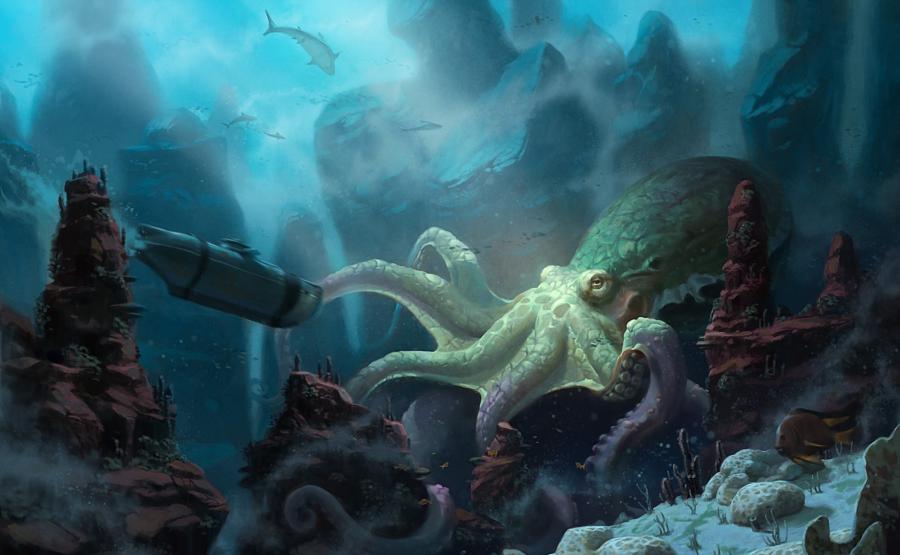This digital illustration depicts an underwater fantasy scene with an enormous octopus as the central focus. The octopus is positioned on the right side of the image, with its bulbous head and part of its body hued in bluish-green tones, while its tentacles transition to a lighter palette of white and light purple. The creature's eye is clearly visible, and its body angles toward the upper right.

In the foreground, various forms of sea life, including coral and fish, are evident, along with rocky outcroppings of maroon and white sediment. These rocky formations add depth to the landscape, appearing in both the immediate and distant background. 

Towards the left side of the scene, a man-made submarine is approaching the massive octopus at a moderate pace, though its size is minuscule in comparison. The submarine, slightly blurry as if in motion, directs the viewer's attention towards its destination. 

A prominent beam of light cascades from the top left of the image to the bottom right, illuminating the giant octopus and adding drama to the composition. In the background, towering rock formations that resemble pointy castles add to the fantastical ambiance.

Furthermore, a few great white sharks swim distantly at the top of the image, appearing both small in comparison to the submarine and the colossal octopus. The intricate details create a vivid and immersive underwater world, blending elements of realism with fantasy.